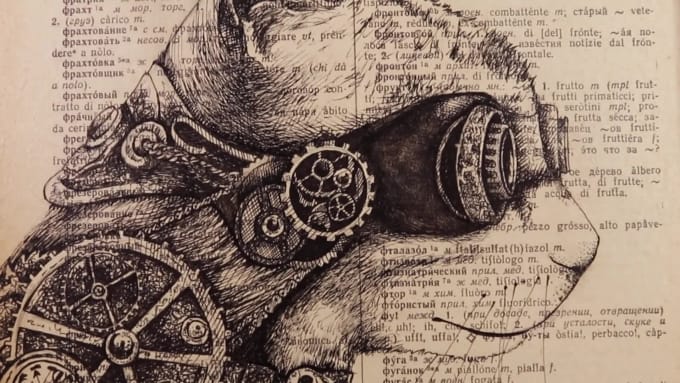This image features a meticulously detailed ink drawing of a cat, executed in a steampunk style. The feline appears against a backdrop of what seems to be a foreign language dictionary page, possibly Russian. The cat, or otter as one might mistake it for, is adorned with antique-looking goggles, intricately attached to its head with a headband-like apparatus. These goggles, along with several gears depicted both within and around them, emphasize a theme of invention and mechanical tinkering. The cat's expression is contemplative, gazing off to the side, which adds an element of curiosity and depth to the portrait. The combination of the shaded pen work and the mechanical elements intricately integrated into the animal's headwear showcases the artist's technical prowess and creativity.